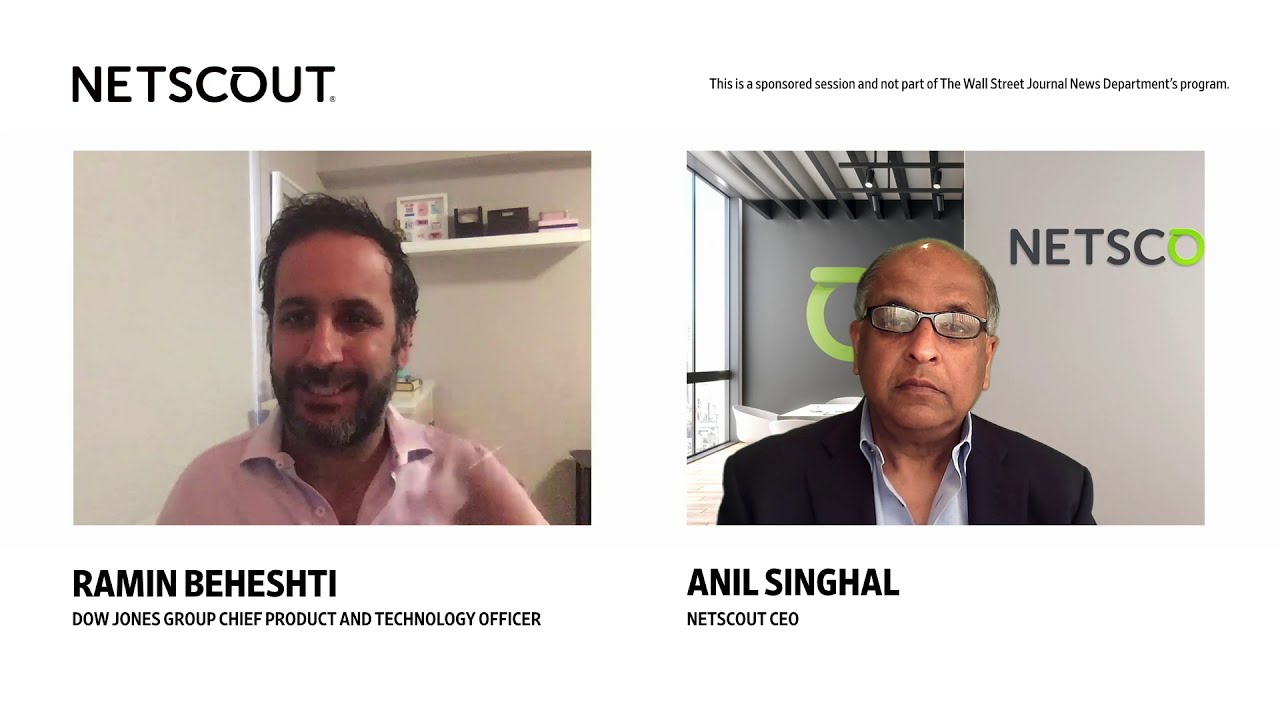This photograph showcases two individual headshots on a white background, likely representing participants in a conference call. The image is divided into two sections: on the top left, the text "NetScout" is displayed in black, while a note on the top right clarifies that it is a sponsored session not affiliated with the Wall Street Journal News Department program.

On the left side, a headshot of Raman Behishti is featured. He has short black hair, a mustache, and a beard, and is dressed in a button-up, collared shirt, which appears to be pink. Behind him are shelves adorned with knickknacks, placing him in what could be an office or bedroom. Above his image, the text "NetScout" is displayed in all caps, and below it, his name, "Raman Behishti," is printed along with his title, "Dow Jones Group Chief Product and Technology Officer."

On the right side, another headshot shows Anil Singhal, a man with balding gray hair on the top but short hair on the sides and back, and he wears narrow glasses. He is dressed in a suit and appears to be in a NetScout office, evidenced by the partial company logo "NetSco" visible behind him. Below his image, his name, "Anil Singhal," is displayed along with his title, "NetScout CEO," all in black text.